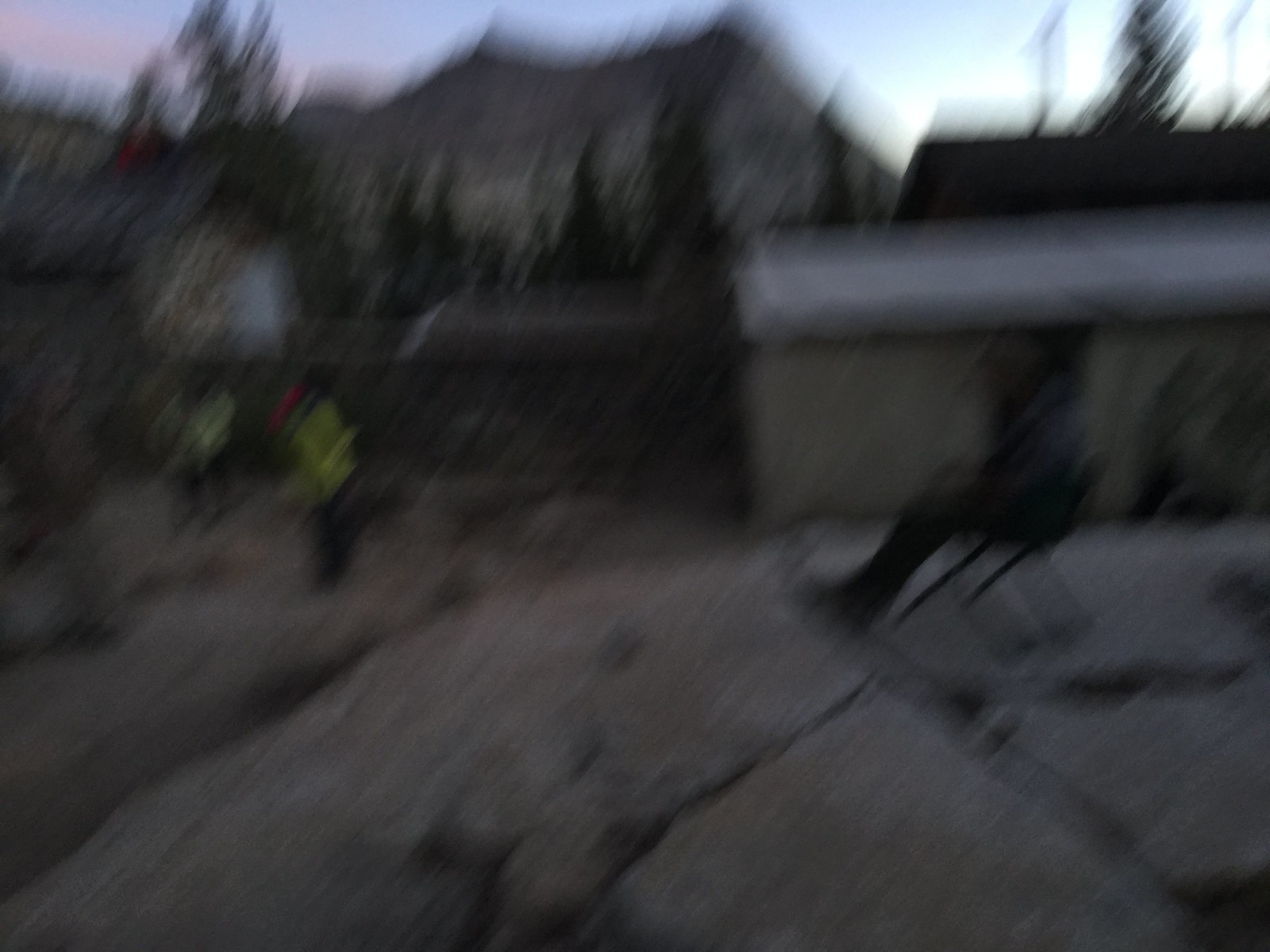In this very blurry photograph, two men are seen working outside amid what appears to be a heavy snowfall. The scene seems to be set either at dawn or dusk, judging by the varying hues in the sky. They appear to be shoveling snow, with visible snow drifts accumulating in the foreground. In the background stand some low, utility-like sheds, one of which has snow atop its roof. Evergreen pine trees are discernible beyond the sheds, their green contrasting with an arid, earthen-colored mountain range in the distance. The man on the right is dressed in a yellow coat and a red hat, while his companion on the left, who is shoveling, is in a cream-colored coat and a dark hat. The sky in the far background displays a beautiful palette, with pink shades to the left and brighter tones indicative of either a sunrise or sunset to the right.